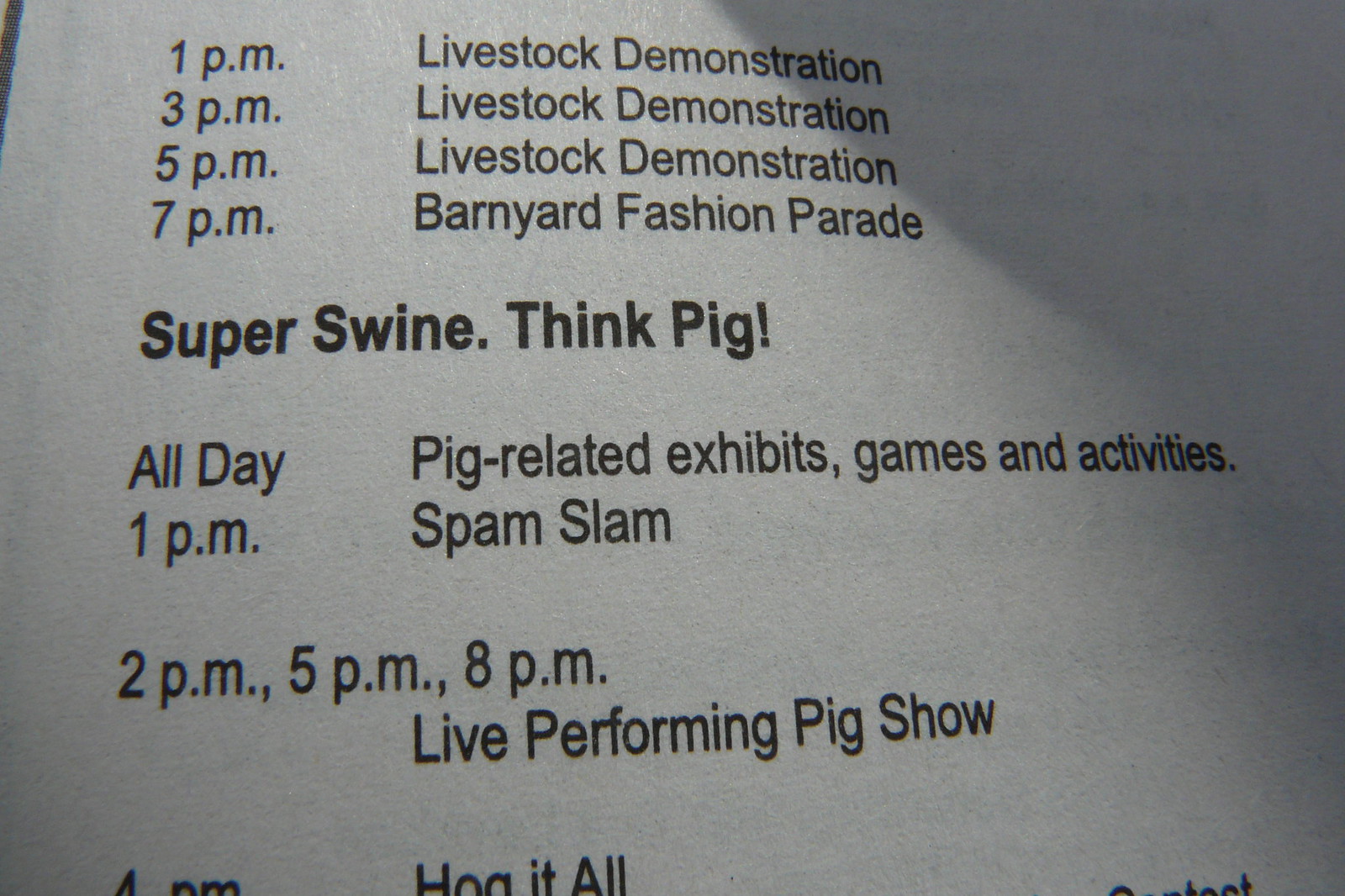This photograph features a white printed page with black text, partially obscured by shadows, particularly in the upper right corner. The page appears to be an announcement for events at a fair, starting with a schedule of livestock demonstrations at 1 p.m., 3 p.m., and 5 p.m., followed by a Barnyard Fashion Parade at 7 p.m. The middle of the page prominently displays the title "Super Swine - Think Pig," indicating an all-day event focused on pig-related exhibits, games, and activities. Specific events under this theme include a Spam Slam at 1 p.m., and Live Performing Pig Shows at 2 p.m., 5 p.m., and 8 p.m. Partially obscured text suggests another event at 4 p.m., possibly titled "Hog It All."